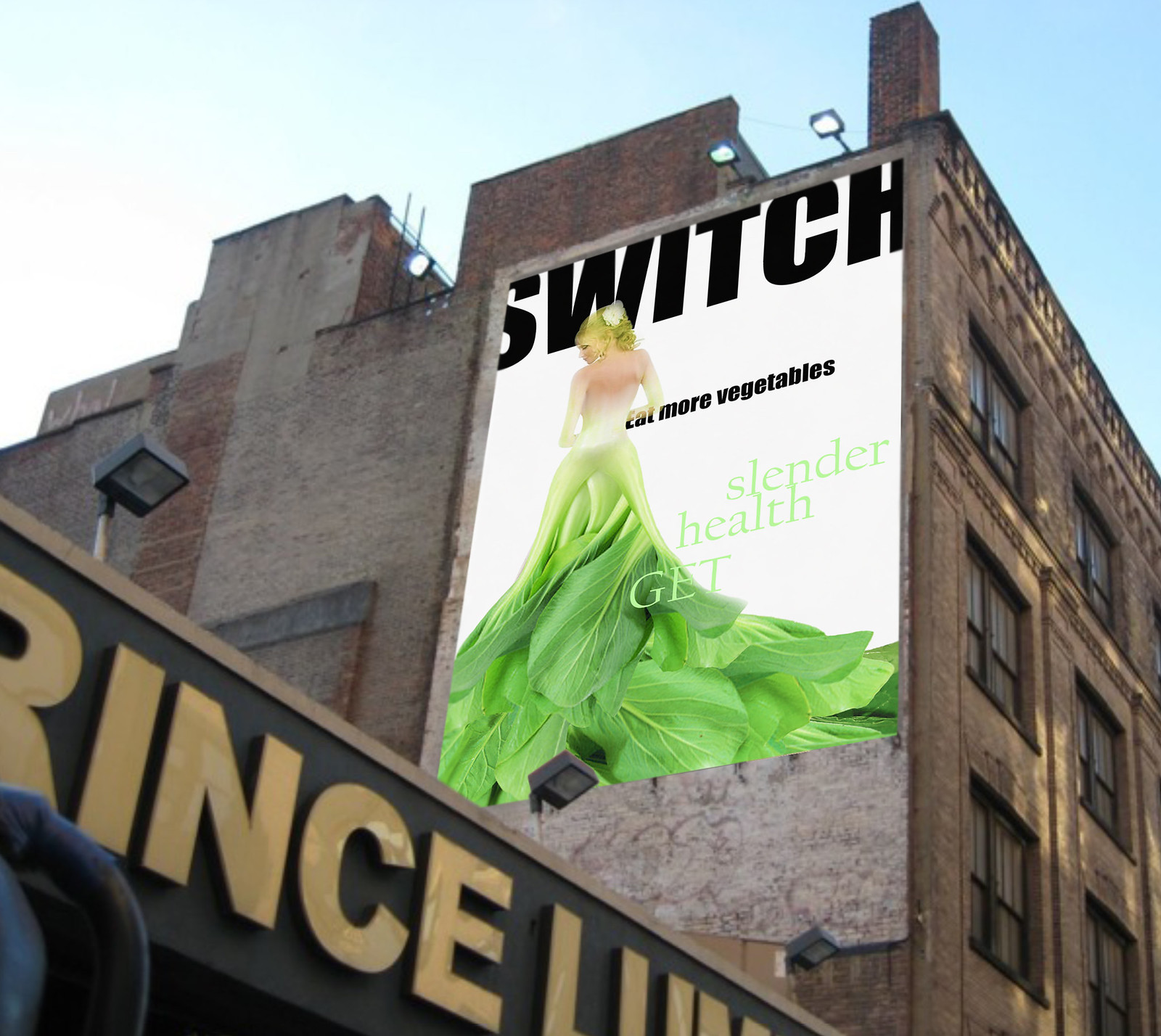The image is a high-quality photograph taken from the ground, depicting a mock-up of a future billboard on the blank side of a building. The angle allows us to see the broadside, rather than the street-facing side, of the structure. This side is devoid of windows, contrasting the front-facing side, which features numerous windows overlooking the road. The mock-up billboard appears perfectly lit without any shadows, indicating it is digitally imposed rather than physically present. The billboard showcases a message encouraging healthier eating habits: "Switch. Eat more vegetables. Slender Health Kit." It features an image of a woman seen from behind, adorned in a large, leafy dress. To the lower left of the scene, the roof of a much shorter building is visible, displaying partial lettering that reads "R-I-N-C-E-L-I" before being cut off, making it difficult to discern the full name, possibly "Prince Line" or "Prince Link." This image provides a clear and detailed vision of what the future billboard could look like once installed.